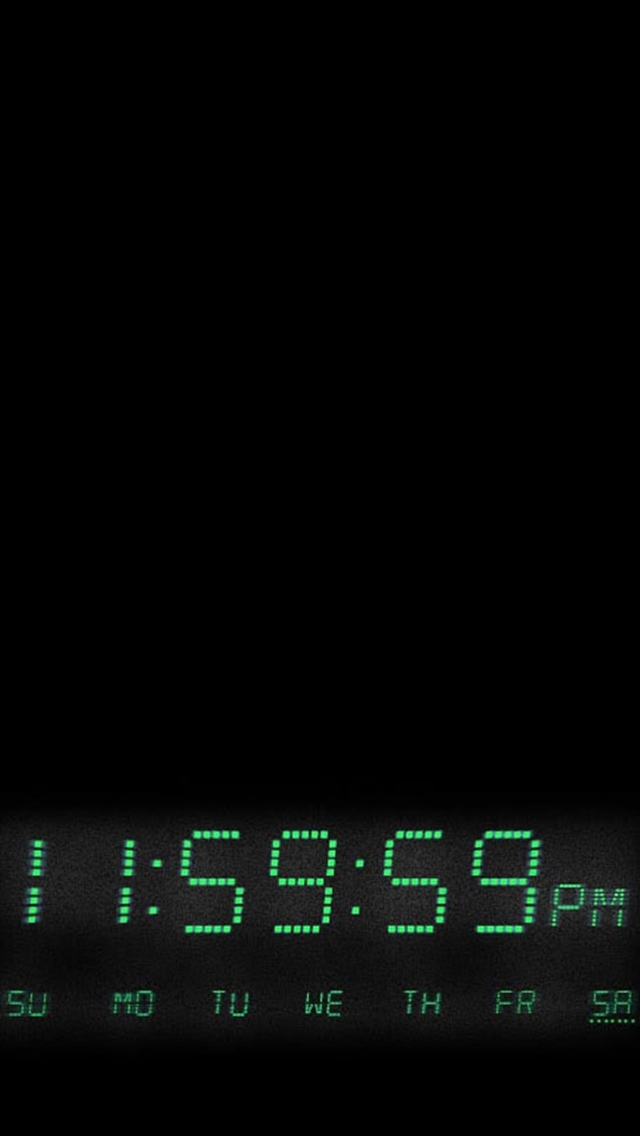The image features a digital clock set against a flat black background, reminiscent of a potential lock screen for a smartphone or tablet due to its sleek, minimalist design. The top four-fifths of the image is blank, emphasizing the clock at the bottom. The clock display has a slightly lighter gray background compared to the rest of the image. The time is shown as "11:59:59 PM" in a green, dotted font, where each numeral is formed by a series of illuminated dots, giving it a digital, pixelated appearance. Below the time, there are abbreviations for the days of the week (SU, MO, TU, WE, TH, FR, SA) with "SA" being underlined with dots, indicating it is currently Saturday. The overall aesthetic of the clock—with its green digits against the black backdrop—evokes a certain futuristic, almost Matrix-like feel.